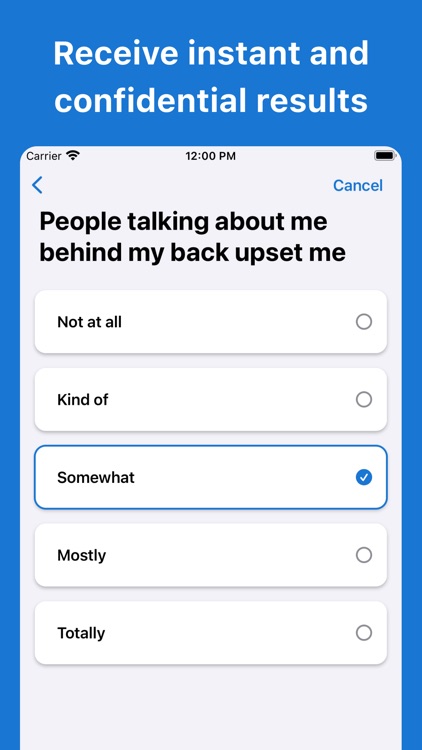The image is a screenshot emulating a mobile phone display set against a blue background. The central focus is the simulated phone screen, which has a light gray background. 

At the top of this screen, in bold white text on a blue banner, it reads, "Receive instant and confidential results." Below, the UI of the simulated phone is depicted with typical elements: the text "Carrier" on the left, a Wi-Fi symbol, the time "12:00 PM" in the center, and a battery icon on the right.

Directly beneath this top banner, there's a navigation bar featuring a left-pointing caret in blue on the left and a "Cancel" button on the right. Below this, in bold black letters, is the statement, "People talking about me behind my back upsets me."

Beneath the statement are five horizontally aligned, rounded rectangle buttons, each representing a different response level: "Not at all," "Kind of," "Somewhat," "Mostly," and "Totally." To the right of each option is a circle where users can indicate their selection. The option "Somewhat" is selected, highlighted in blue with a white checkmark inside the circle.

The phone display design continues with the light gray and blue background extending towards the edges, but the image cuts off before reaching the bottom of the simulated phone display, omitting any view of a home button or additional controls.